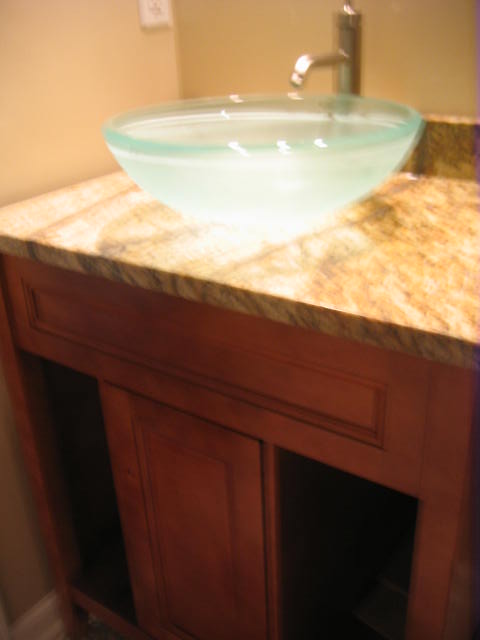This vertically-oriented photograph captures a slightly blurred image of a sophisticated bathroom vanity. The vanity features a medium-colored brown wooden base with a distinguished marble countertop that showcases a delicate blend of cream and brown hues. Atop the marble sits a modern, clear glass bowl sink paired with a sleek silver faucet, though the water flow is indiscernible due to the blur. The backdrop of the vanity is a camel-colored wall with a strip of marble running horizontally along the back, harmonizing with the countertop. The base of the vanity includes two wooden paneled drawers designed to slide rather than open and close traditionally; they are currently positioned partially open, with one panel overlapping the other. In the far left corner of the image, a piece of white floor molding can be seen, adding a touch of contrast to the scene.